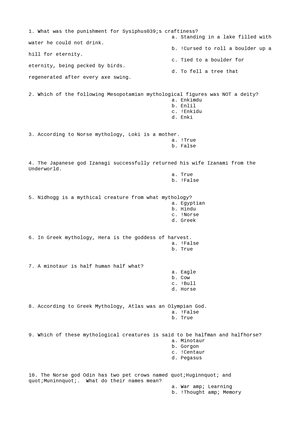This image is a screenshot displaying a questionnaire. The background of the image is white, and the text, which is rendered in an extremely small font likely around 6 points or less, is difficult to read without magnification. The questionnaire is organized with questions numbered from 1 to 10. Each question is followed by multiple-choice answers. While most of the questions offer four possible answers to select from, three specific questions provide only two possible answers, which are true or false options. Due to the minuscule font size, the content of the questions and answers cannot be clearly discerned, though occasional words can be picked out here and there. The overall structure and layout suggest a standardized format, but the overly small text size renders it nearly unreadable in this screenshot.